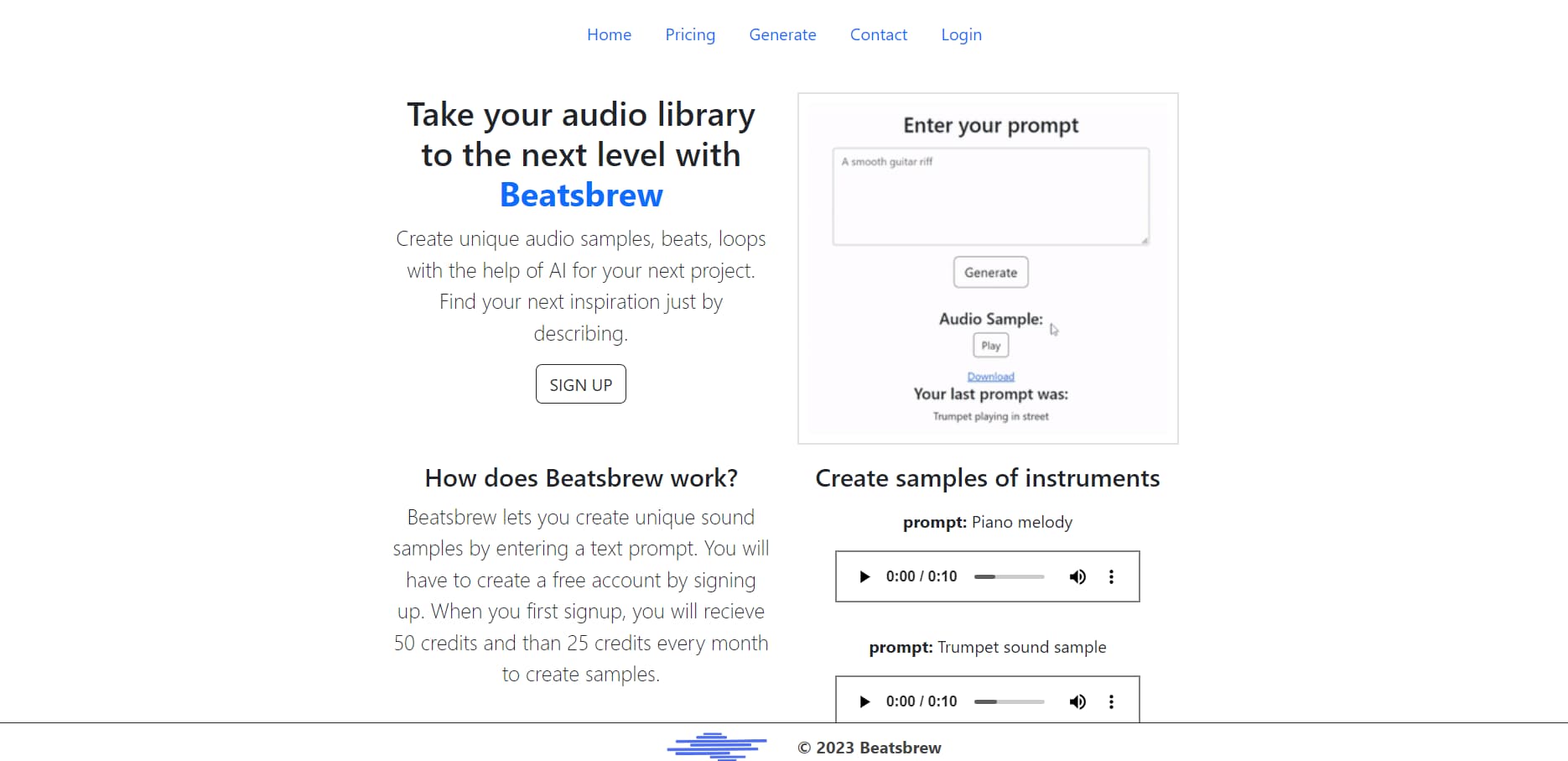**Caption:**

Advertisement for Beats Brew

At the top of the image, the navigation menu features links to Home, Pricing, Generate, Content, Contact, and Login. On the right-hand side, there's a prompt entry box where users can input text to generate audio samples or upload their own audio files. The advertisement highlights the tagline, "Take your audio library to the next level with Beats Brew. Create unique audio samples, beats, and loops with the help of AI for your next project. Find your next inspiration just by describing it."

Users are invited to sign up for a free account to access the platform. Upon registration, new members receive 50 credits and then 25 additional credits each month to create sample tracks. The platform supports generating unique sound samples by entering text prompts. Examples provided include a piano medley and a trumpet sound sample, each lasting about 10 seconds. At the bottom, it is noted that the website and information are up-to-date as of 2023.